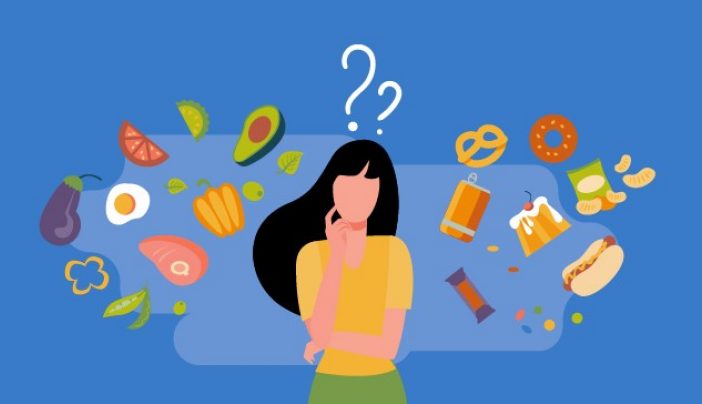The image depicts a graphic illustration of a faceless woman with long black hair, styled with bangs and flowing behind her shoulders. She is light-skinned, possibly Caucasian or Asian, dressed in a yellow short-sleeve top and cropped green bottoms, likely pants or a skirt. Her left arm is crossed over her waist, while her right elbow is bent, with her hand holding her chin in a contemplative pose. Hovering above her head are two white question marks, emphasizing her indecision. The background is entirely blue, creating a stark contrast with the multitude of food items surrounding her, suggesting she is contemplating her dietary choices. On one side, there are various junk foods such as a hot dog with mustard, a pretzel, a donut, chips, and soda. On the other side, healthier options are depicted, including a halved avocado, a fried egg, a slice of tomato, an eggplant, a yellow bell pepper, a lime slice, and a couple of leaves, along with watermelon, grapefruit, a steak, and carrots. The detailed arrangement highlights the woman's internal debate over choosing between indulgent snacks and nutritious foods.